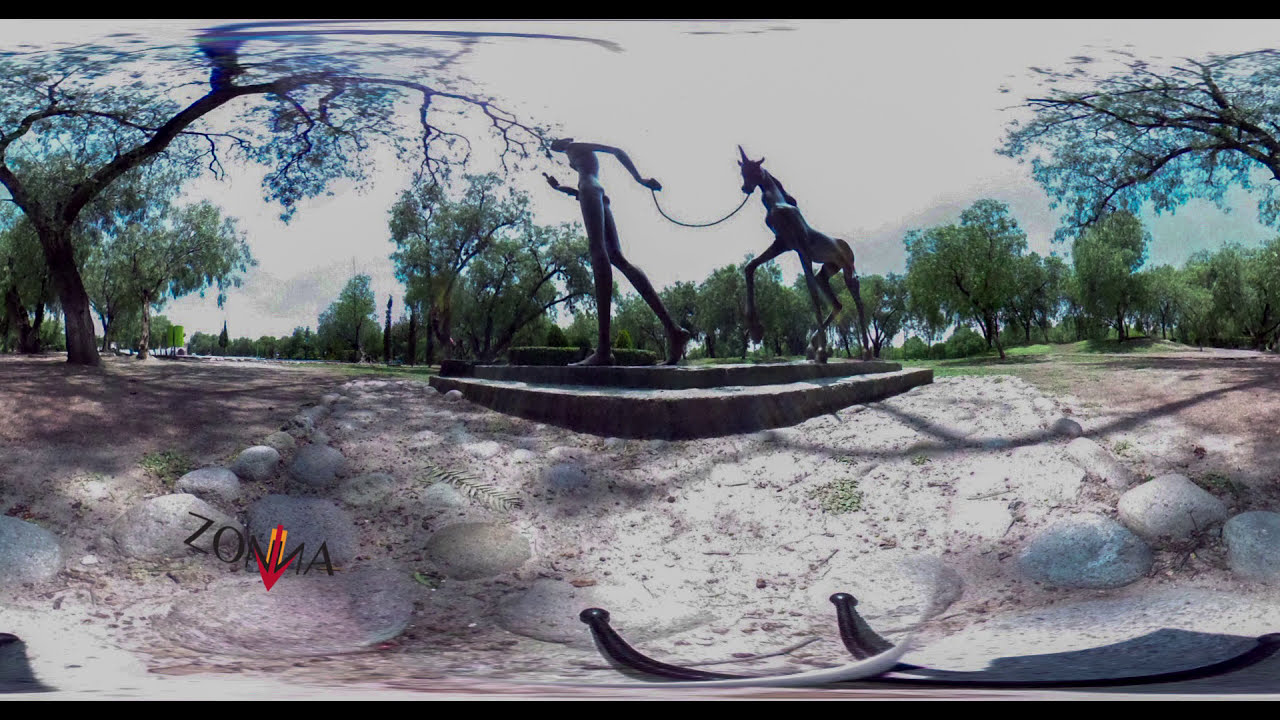The image portrays a panoramic photograph of a public park, characterized by noticeable distortions likely caused by a 360-degree camera. Dominating the center is a striking statue on a small platform: an exaggeratedly tall figure, appearing to be made of metal or rock, with outstretched arms tethered to a unicorn-like creature featuring long slender legs. Surrounding the statue are stone walkways and steps, with trees and green grass filling the background. This panoramic effect warps elements such as a tree branch on the left side, making it reappear on the right. In the bottom left corner, there's the word "Z-O-N-N-A" – one 'N' is reversed – shaped like a down arrow in red against an orange background. The scene is bathed in daylight, revealing a bright sky overhead.